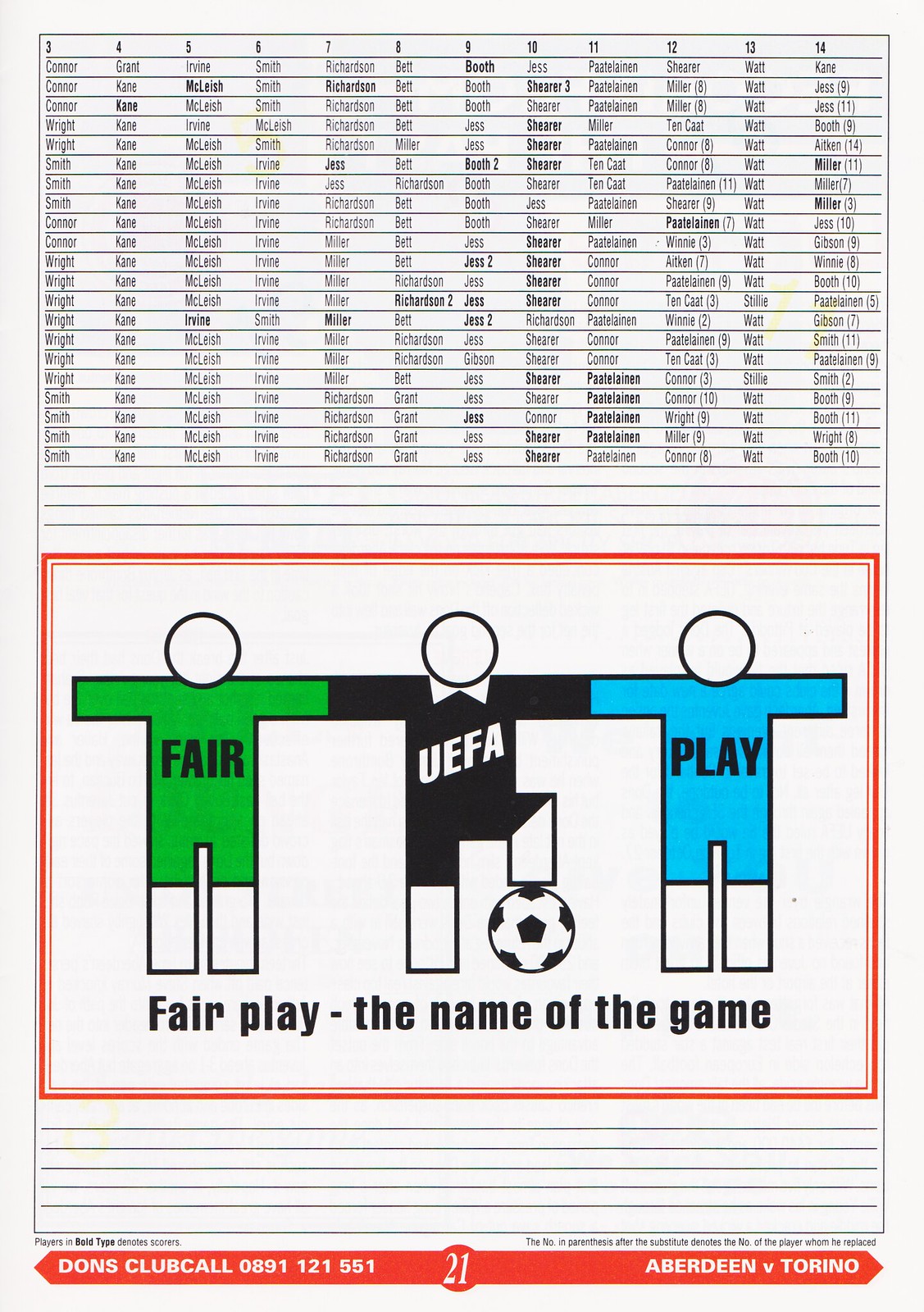The image is portrait-oriented and divided into two distinct halves. The top half features a detailed spreadsheet resembling a player sheet for soccer or football. This spreadsheet has 11 columns and around 15-20 rows, filled with names such as Connor, Grant, Irvine, Smith, Richardson, Bett, Booth, Jess, Pantelainen, Scherer, Watt, and Kane, among others. The columns are numbered from 3 to 14 at the top. The bottom half showcases an advertisement with three stick-figure soccer players holding hands, each wearing different colored jerseys. The first figure, dressed in green, has "FAIR" written on the shirt; the middle figure in black with "UEFA" in white lettering, is stepping on a black-and-white soccer ball; and the last figure, in light blue, has "PLAY" printed on the jersey. Below these figures, there is a caption in black ink reading "FAIR PLAY - the name of the game." Additionally, at the very bottom of the image, there is a red banner with white text that reads "DONS CLUB BALL 0891 121 551," alongside the match announcement "Aberdeen versus Torino" in white text.